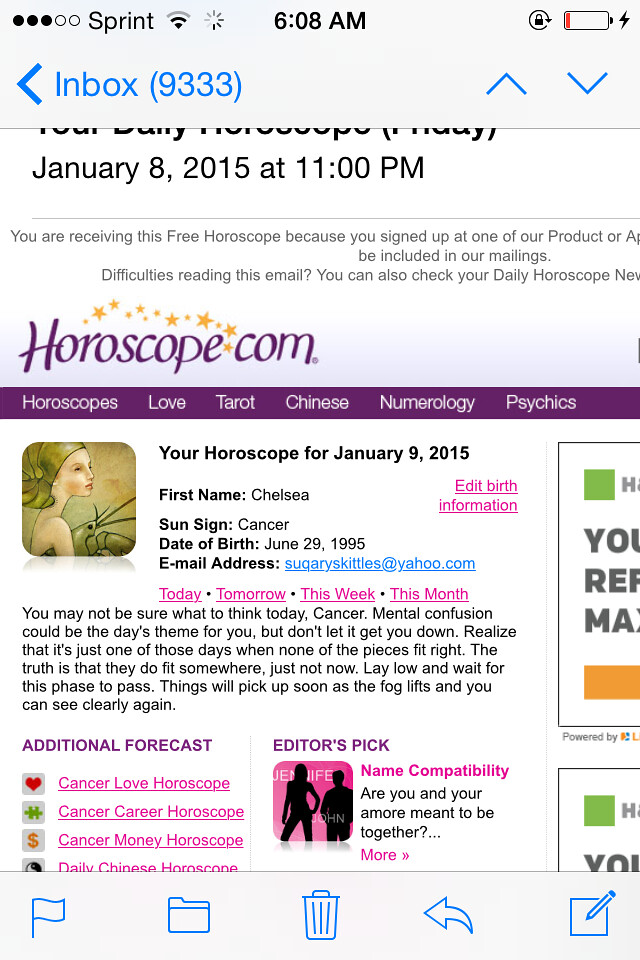A detailed screenshot of an email displayed on a cell phone screen, featuring a horoscope from Horoscope.com. In the top left corner, there are five dots indicating signal strength, with three filled and two empty. Next to it, the word "Sprint" signifies the service provider. Adjacent symbols include a Wi-Fi icon, a spinning gear for loading, a lock icon with a circular border, and a battery icon showing a red line indicating low charge, accompanied by a black lightning bolt.

Centered at the top, the time reads "6 to 8 a.m." Below "Sprint" is the word "Inbox" in blue, with a left-pointing arrow and the number (9333) in parentheses. To the left of this, there are blue up and down arrows for navigation within the inbox.

The main body of the email has a timestamp of "January 2015 at 11:00 p.m." It starts with partially visible text, "you're receiving this free horoscope because you signed up for...," followed by further incomplete lines. Below, in purple, "horoscope.com" is displayed with gold stars above it. A purple bar with white text reads "horoscopes, love, tarot, Chinese, numerology, physics."

To the left, there is a square image of a hand-drawn face turned to the right, with a green head covering and a brown, leafy background. Beside it, the personalized horoscope states "Your horoscope for January 9, 2015," addressing Chelsea, a Cancer born on July 29, 1995, with the email "sugarskittles@yahoo.com." An "edit birth information" link follows.

In pink text, the options "Today, Tomorrow, This Week, This Month" are listed. Below is a paragraph of black text, followed by two columns with additional forecasts: "Cancer love horoscope, Cancer career horoscope, Cancer money horoscope, Daily Chinese horoscope," each accompanied by a small gray box.

An "Editor's Pick" section features "Name compatibility" and a query "Are you and your mate meant to be together?" with the acronym "MRE" beneath it. This section includes a gray rounded square with a silhouette of a man and woman.

At the bottom of the screen, a gray bar with various icons appears: a blue flag, a folder, a trash can, a reply arrow, and a compose icon. The layout reflects typical email functionalities within a mobile device interface.